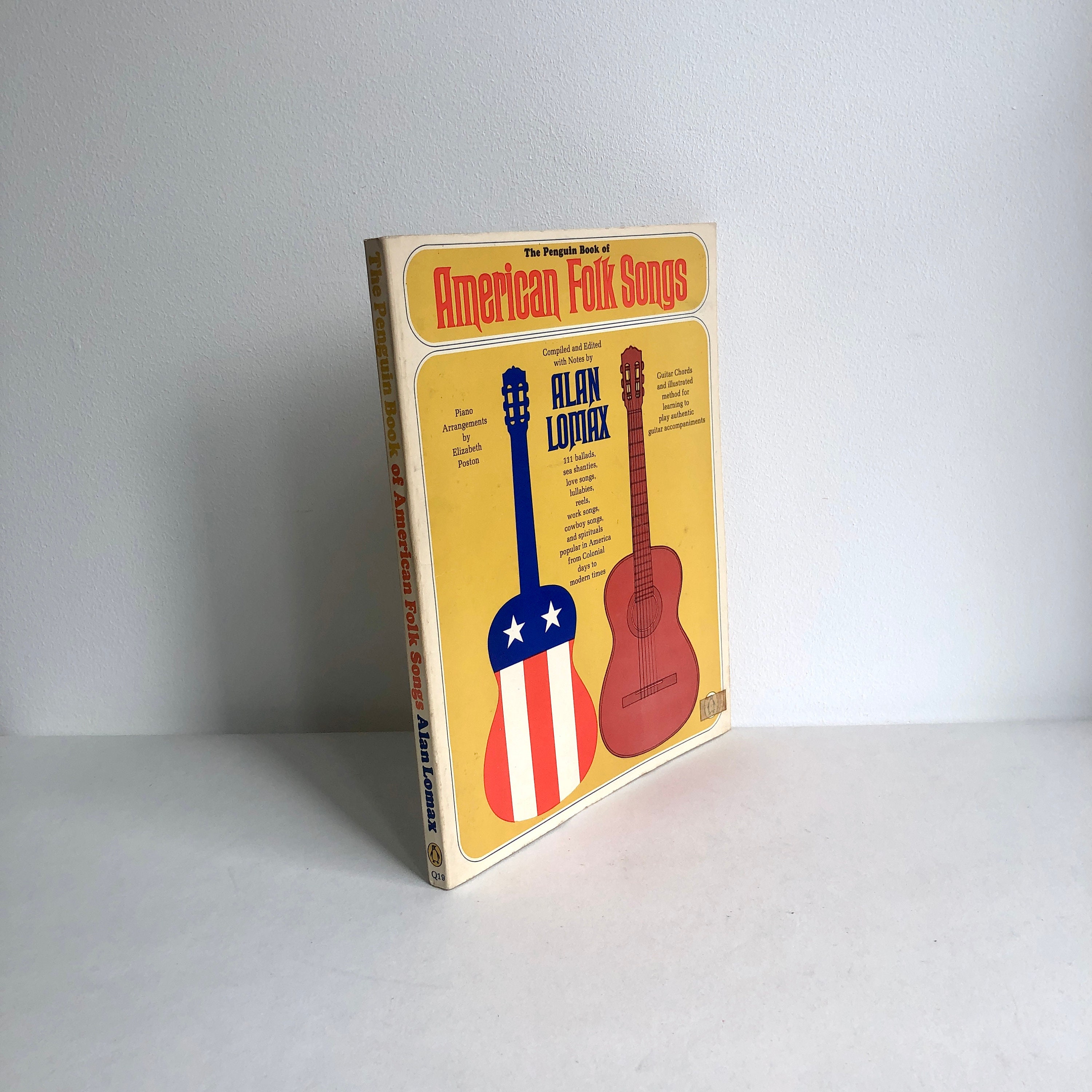The image depicts a vintage, weathered item, likely from the 1960s or 70s, that appears to be a thin cardboard case, possibly housing a record or book titled "The Penguin Book of American Folk Songs" by Alan Lomax. The case, oriented vertically, features a predominantly yellow and off-white color scheme with "American Folk Songs" prominently displayed in red within a circular yellow backdrop. The cover art includes two side-by-side guitars: the left guitar is emblazoned with an American flag motif, featuring a blue neck with two stars and red and white stripes on the body, while the right guitar is a classic brown acoustic. The background of the image itself is flat and white.